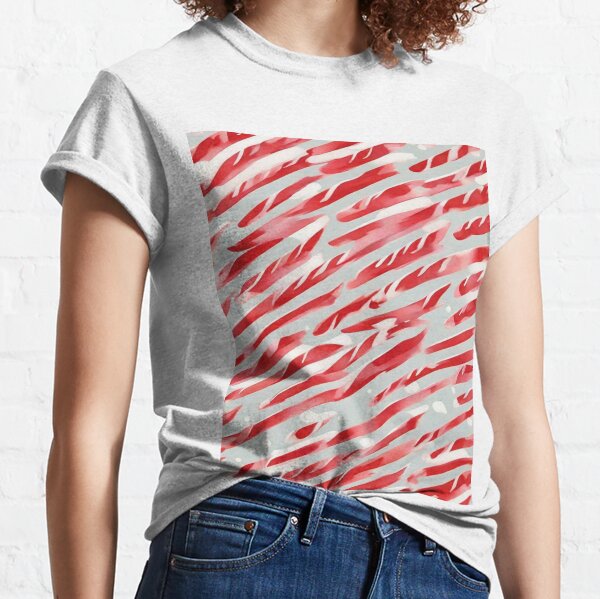This photograph features a female model, identifiable by her curly red hair, against a white painted brick wall. The model, whose face is not visible, is showcasing a white short-sleeved t-shirt with rolled-up sleeves and a unique graphic on the front. The t-shirt prominently displays a large rectangular design comprised of red and white stripes, with some pink hues interwoven among the stripes. The stripes are primarily diagonal, running from the bottom left to the top right. One side of the t-shirt is casually tucked into the top of her blue jeans, specifically on the right side. Her arms hang naturally at her sides, and while you can discern her fair skin and a bit of her hair, the overall image focuses on the clothing, highlighting the relaxed yet stylish presentation of both the t-shirt and jeans.